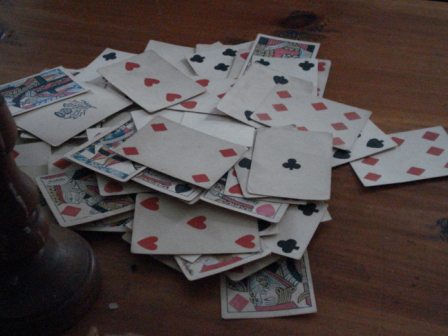A dark, moody photograph showcases a scattered pile of playing cards on a natural wood table. Among the visible cards, an ace of clubs, a four of diamonds, and a complete three of diamonds stand out. The composition includes partial glimpses of a five of hearts, an eight of diamonds, a jack, a king, and possibly a five of clubs. The cards are from all four suits—hearts, clubs, diamonds, and spades—distinguished by their red and black colors. The card backs display intricate, detailed patterns in blue, red, and white hues, typical of a standard deck. The left side of the image is notably darker, suggesting the presence of an object like a lamp that casts a shadow. The natural wooden table adds a rustic contrast to the otherwise dark scene, which lacks any true white tones, contributing to the overall somber atmosphere.